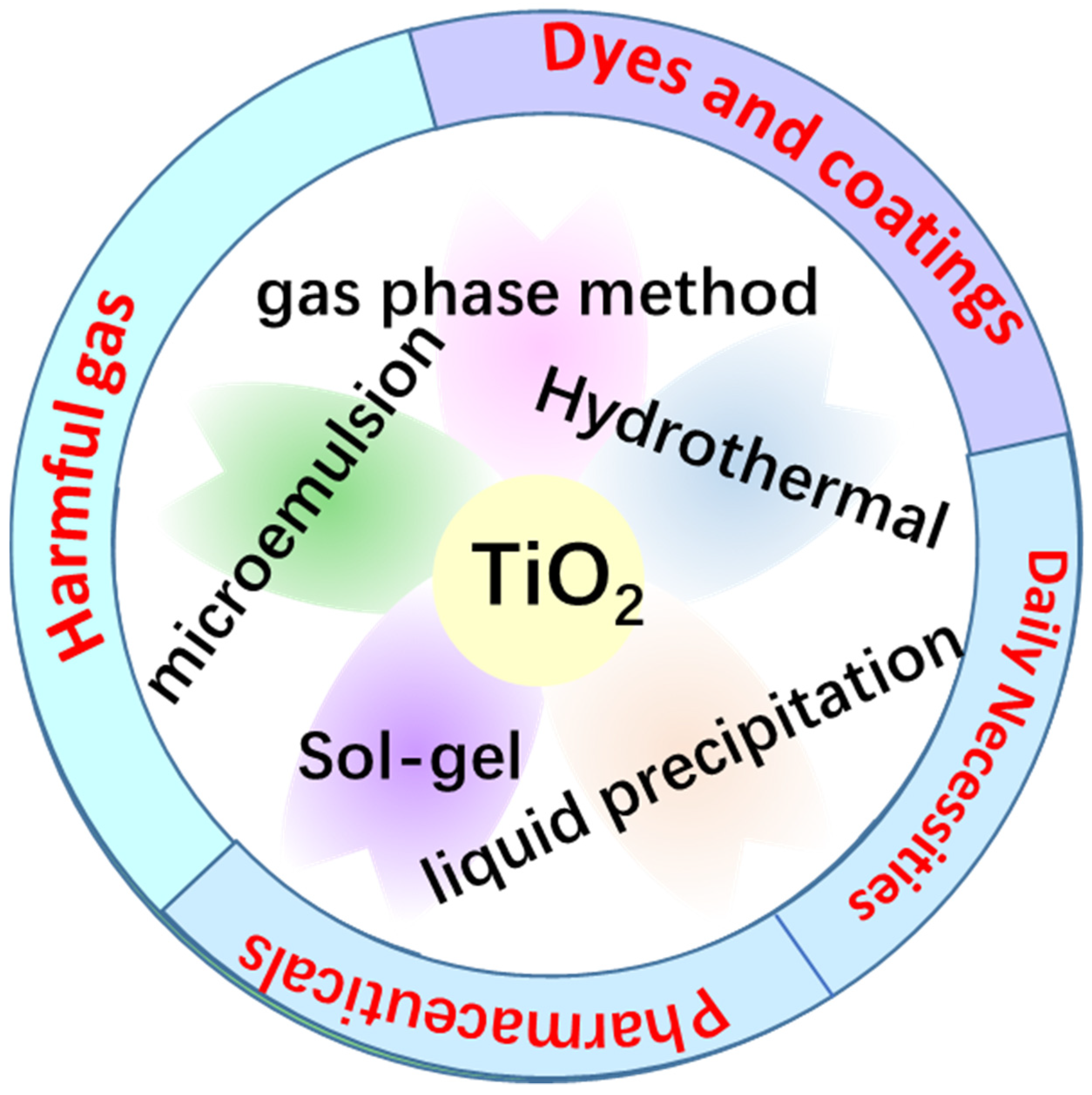This illustration is a color diagram from a textbook, likely pertaining to a scientific or chemical subject such as biology or organic chemistry. The image features a large circle with a smaller circle inside it. Around the outer edge of the larger circle, written in red letters, are the categories "harmful gases," "dyes and coatings," "daily necessities," and "pharmaceuticals," arranged in a clockwise fashion. The smaller inner circle contains black text that lists various methods: "gas phase method," "microemulsion," "hydrothermal," "liquid precipitation," and "Sol-gel." At the very center, within a yellow circle, is the chemical formula "TiO2." The background features a faint, pastel-colored flower shape with five petals in shades of purple, green, and blue, adding a light, decorative element to the scientific illustration.